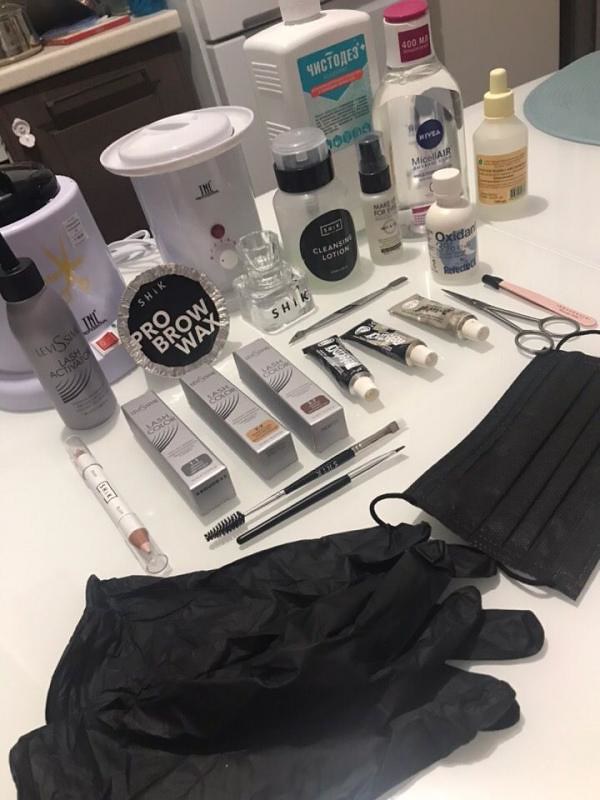A countertop, likely in a kitchen as suggested by the visible refrigerator, cutting boards, and other appliances in the background, is meticulously arranged with a diverse array of beauty products. At the forefront are several bottles containing creams in various sizes, alongside boxes labeled "Lash Color" and "Eyeliner Color," complete with a visible applicator brush. A pen-like object rests to the left of these boxes, while hair-cutting scissors can be seen on the right. Prominently displayed in front are a black surgical mask and a pair of black gloves. 

Towards the back of the setup, larger beauty items come into view: a bottle labeled "Lash Activator," a container for "Pro Brow Wax," and a bottle named "Cleansing Lotion." There’s also a bottle labeled "Oxidant," adding to the extensive assortment.

Among these, one notably large white bottle with a blue label in the back captures attention, uniquely featuring Russian text amidst otherwise English-labeled products. The variety and quantity of items showcase an expansive collection aimed at different beauty needs, creating a comprehensive snapshot of daily beauty essentials.